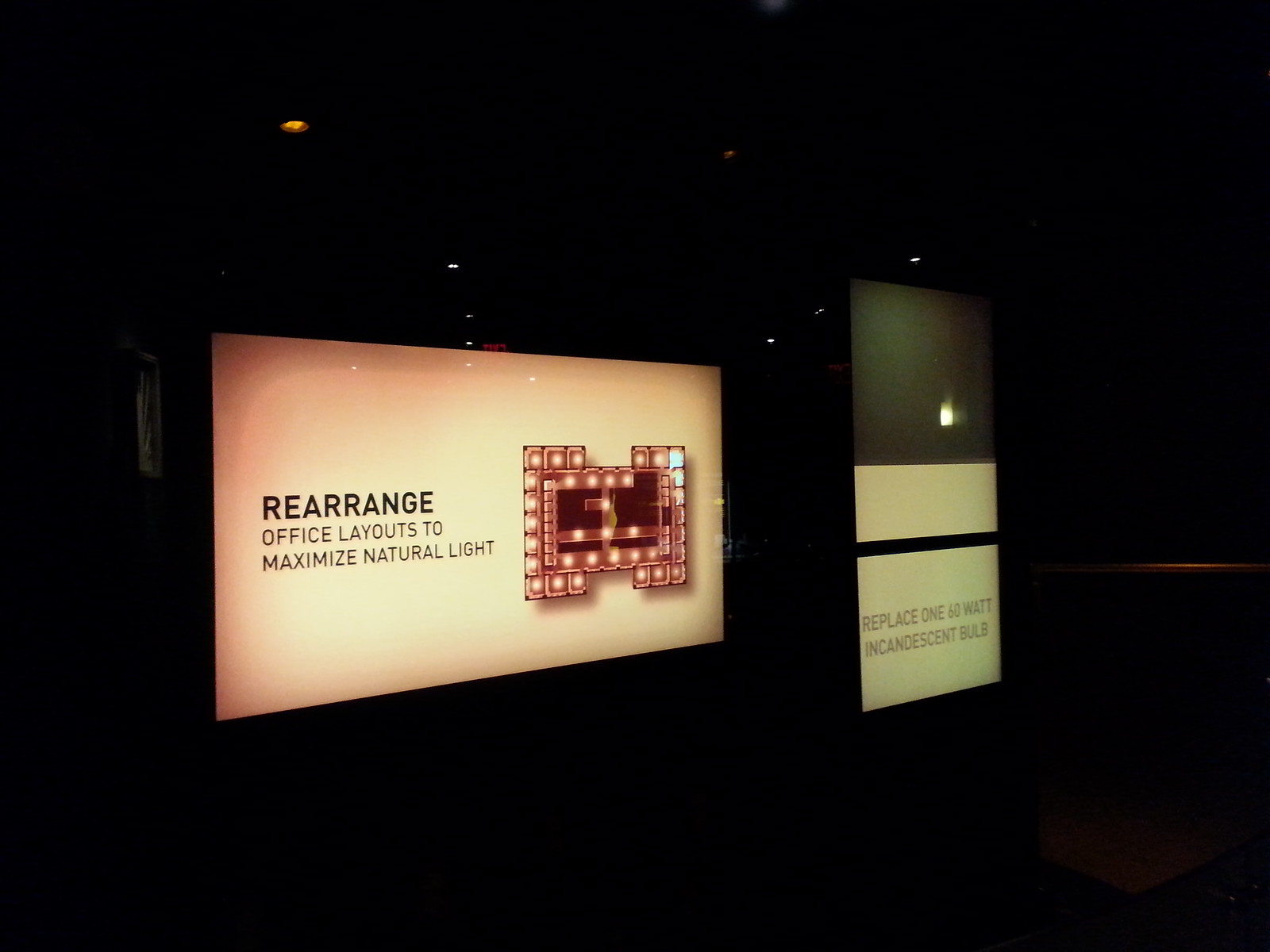The image is a color photograph featuring two illuminated signs against a very dark background, possibly at night or in a dimly lit interior space. The signs are positioned with the horizontal one on the left and the vertical one on the right. The left sign has a pinkish-white background with black text, reading, "Rearrange office layouts to maximize natural light." Adjacent to the text is a diagram resembling an office floor plan with various squares and circular light fixtures. The right sign is divided into two sections: the top portion is gray with a white border and black line, while the bottom portion is white with black text stating, "Replace 160-watt incandescent bulb." In the background, faint recessed lights can be seen, contributing to the overall dark atmosphere of the scene. The predominant colors in the image include peach, burgundy, black, white, and dark green.